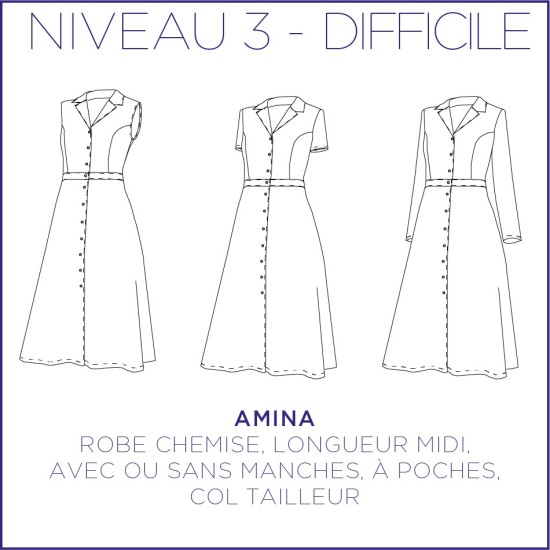The image is an intricate black-and-white sketch depicting three variations of a dress: sleeveless, short sleeves, and long sleeves. All three designs are positioned in a row, outlined with precise blue lines and encased within a thin blue border. Positioned prominently above the dresses in bold purple font is the title "Niveau 3-Difficile." Below each dress design, various descriptive words such as "Amina," "Robe Chemise," "Longueur Midi," and "Avec Poches" are detailed. The entire illustration provides a meticulous and comprehensive look at the different sleeve variations, showcasing the level of detail required for a final piece.